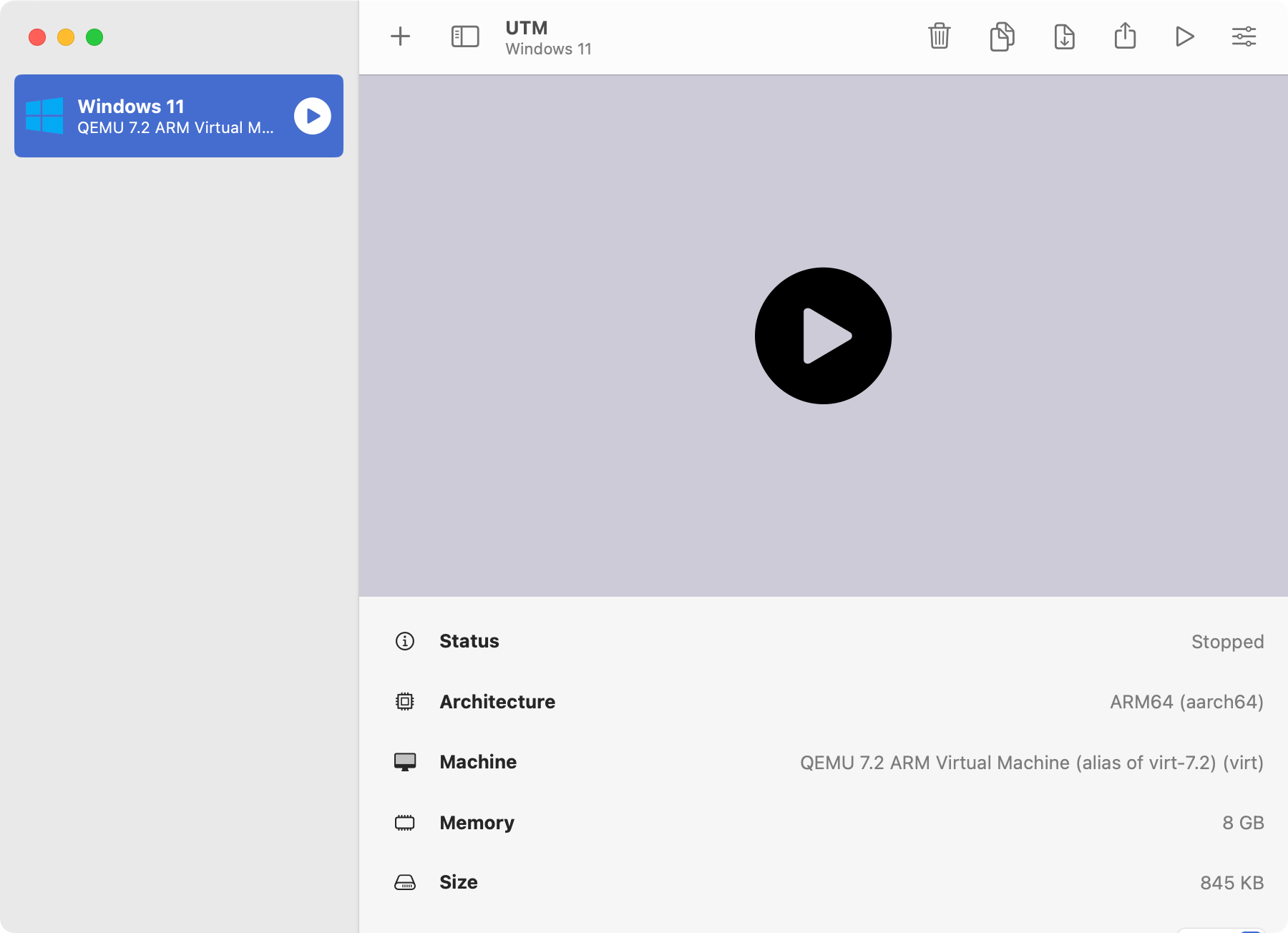This is a screenshot of the UTM display for a Windows 11 virtual machine on a Windows device. The left sidebar features navigation options, while at the top of the main window, a blue header displays the title "Windows 11 QEMU 7.2 ARM Virtual Machine," accompanied by an ellipse with an arrow. Below the header, another section titled "UTM Windows 11" showcases several icons, including trash, copy, download, upload, and an arrow, suggesting various actions that can be performed. In the center, there's a gray square featuring a play icon, indicating a video can be watched. 

Underneath this visual element is a detailed list of the virtual machine's characteristics: 
- **Status:** Stopped 
- **Architecture:** ARM 64 
- **Machine:** QEMU 7.2 Virtual Machine
- **Memory:** 8 gigabytes 
- **Size:** 845 kilobytes